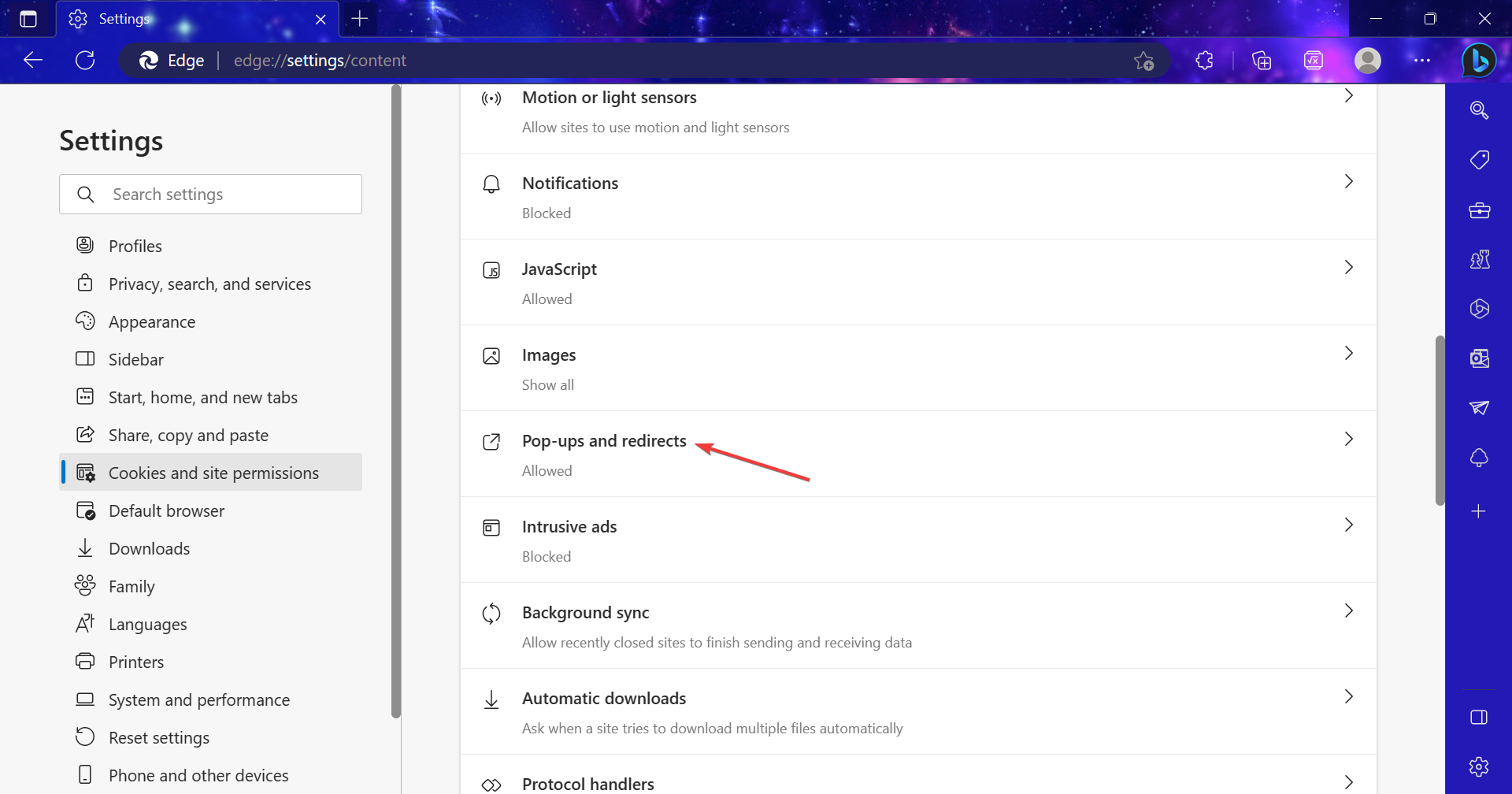The image depicts the settings area of a website, organized with a navigation pane on the left side. This pane contains a series of categories listed in the following order: Profiles, Privacy, Search and Services, Appearance, Sidebar, Start Home, Menu Tabs, Share, Copy and Paste, Cookies and Site Permissions, Default Browser, Downloads, Family, Languages, Printers, System and Performance, Reset Settings, and Phone and Other Devices. The "Cookies and Site Permissions" category is currently highlighted in gray, indicating that this section is open. Additionally, a thin red arrow is prominently pointing towards an option within this section labeled "Popups and Redirects," which is noted to be "Allowed."